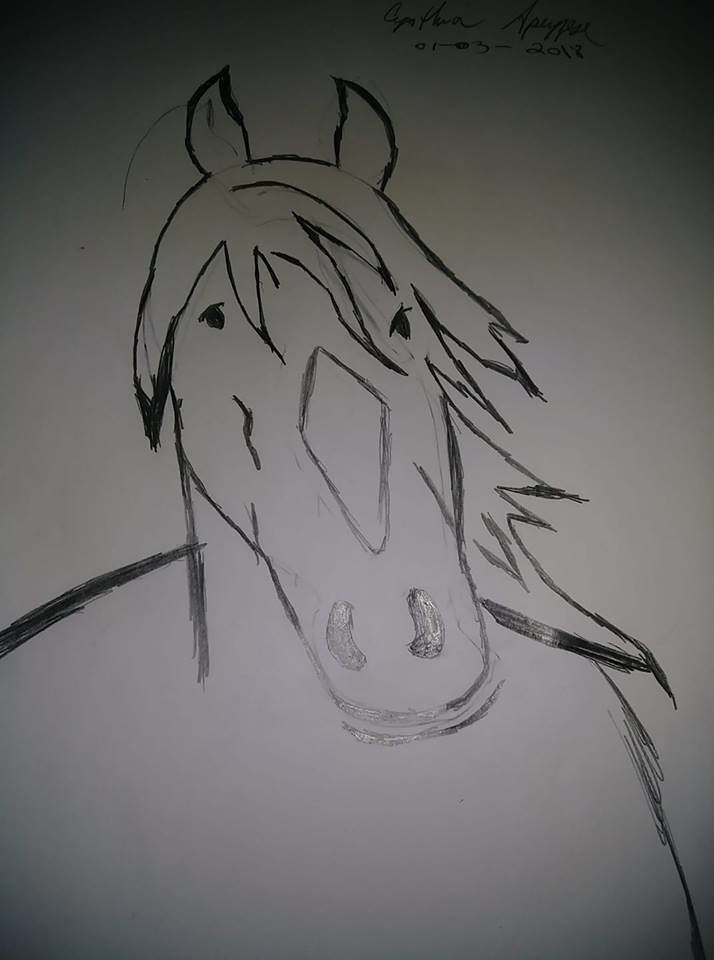This artwork appears to be a detailed pencil or ink drawing depicting the head of a horse merged with a partial human torso. The proportions are noticeably unconventional, adding an abstract or surreal quality to the piece. The horse's head is meticulously rendered, with particular attention given to its nostrils, which appear slightly misaligned. Various markings are present on the horse's face, and its ears and eyes are distinctly drawn. The mane is heavily sketched in black, creating a dynamic sense of movement as it appears to be swept sideways, as if by a gust of wind. The drawing is set against a plain white or gray background, enhancing the prominence of the subject. Notably, there's a small reflective detail near the nostrils. Below the horse's neck, the sketch fades into emptiness, with no further details extending past this point.